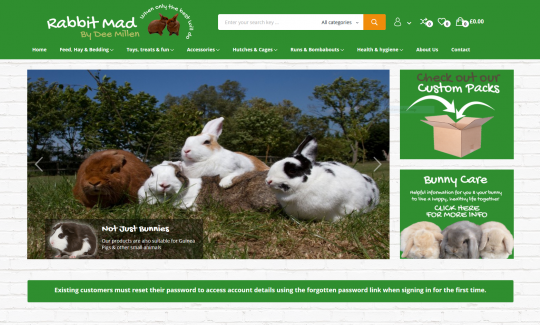This image is a portrait-oriented screenshot of a website titled 'Rabbit Mad' by D. Millen. On the top right, there are images of two small rabbits. In the upper center portion, a search bar is visible with the text "all categories." Below the search bar is a row of tabs, but the text is too small and blurry to read clearly.

Taking up a significant portion of the screenshot is a large image featuring five bunnies in various colors and positions. From left to right, there is a big white and black bunny with numerous black spots, a brown bunny, a white and brown bunny, and a white and light tan bunny that appears to be sitting on another brown bunny facing left. Alternatively, there may be only four bunnies if the second brown bunny is exceptionally large.

At the bottom right corner of the image, the text reads "not just bunnies," while on the right side, there are promotional texts stating "check out our custom packs" and "bunny care. Click here for more info." The context suggests that the website offers products for bunny care, though they do not ship actual bunnies.